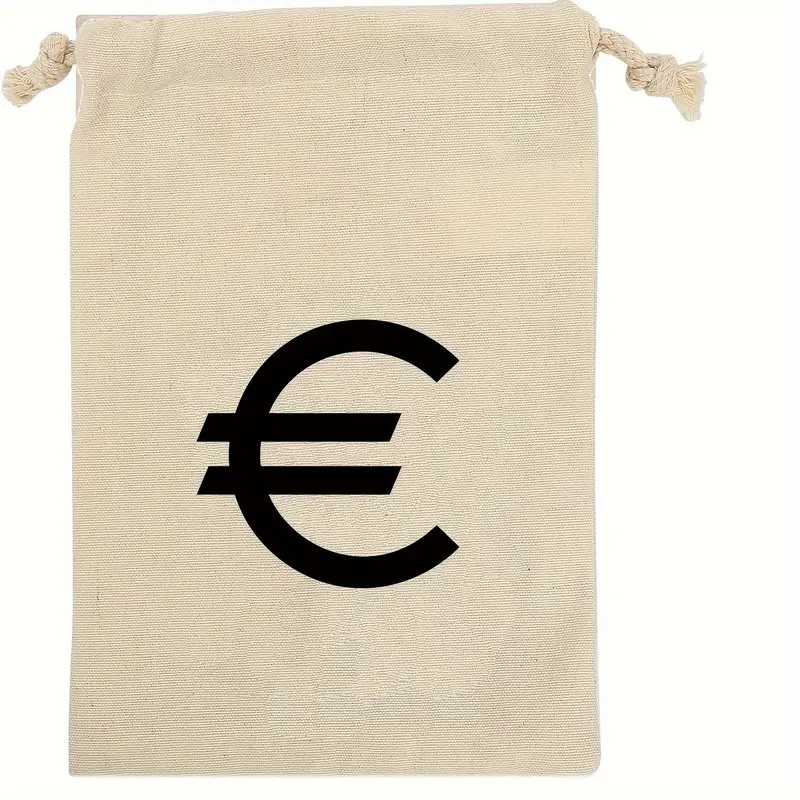The image depicts a small, tan canvas drawstring bag prominently featuring the Euro currency symbol. The symbol, which resembles a capital letter 'C' intersected by two parallel horizontal lines, is printed in black and located in the center of the bag. The top of the bag has a drawstring closure consisting of two tan-colored ropes, each ending in a knot. The strings are not pulled tight, leaving the bag open. The bag is displayed lying flat against a white backdrop.